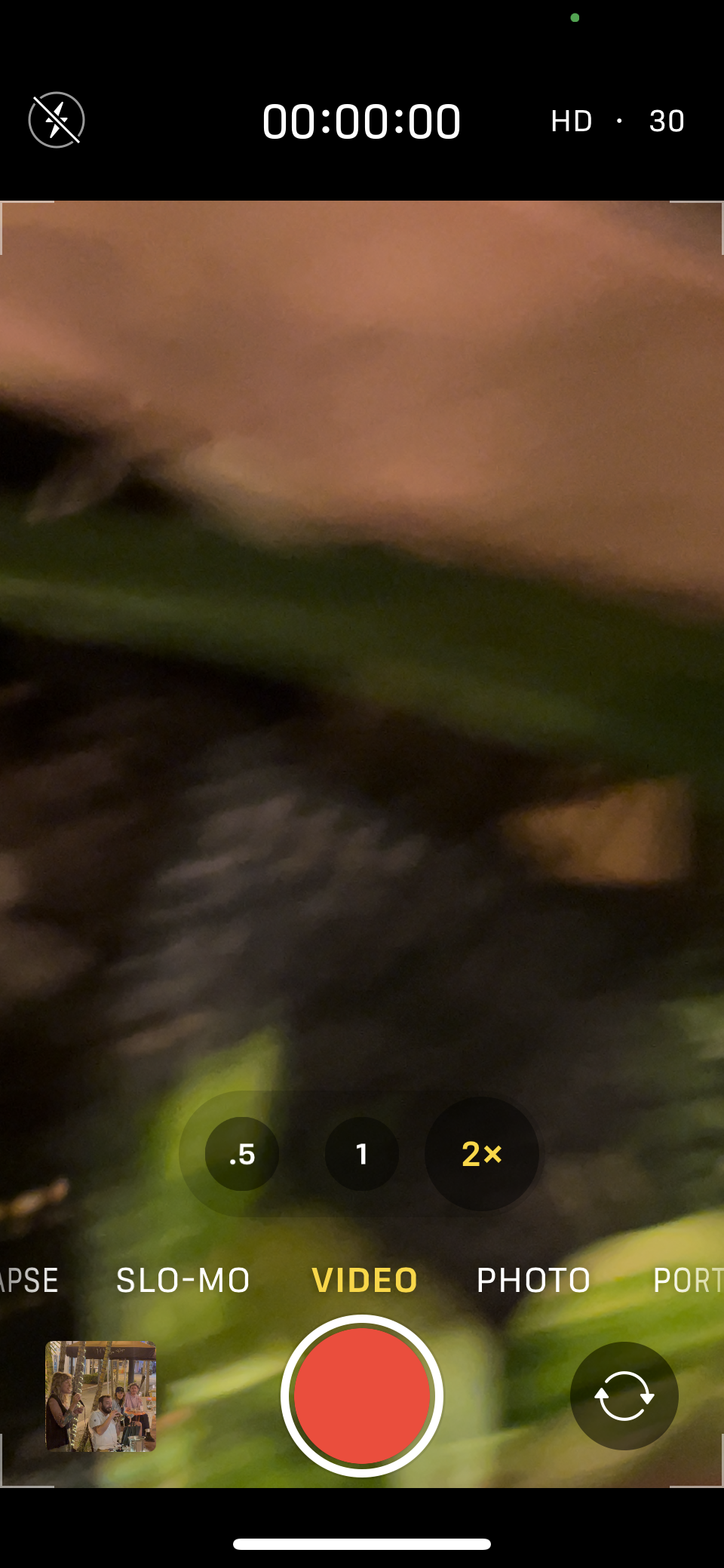A blurred still from a video depicting the top portion of an unidentified animal's head, partially obscured by on-screen controls. The animal, possibly a cat, has eyes that appear green, though the image quality is poor and further details are indiscernible. The upper section of the frame features a nondescript tan color, adding to the overall ambiguity.